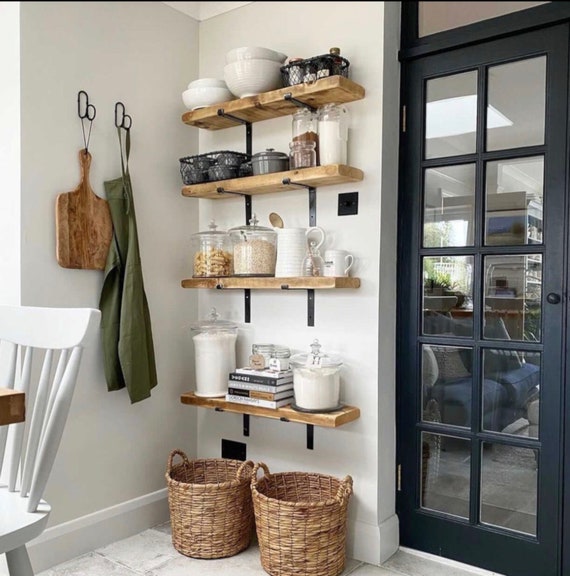The photograph captures a pristine, well-organized kitchen area that gives off a cozy, inviting feel. Dominating the clean, white wall are four neatly arranged wooden shelves, displaying an assortment of dishes and pottery. The top shelf showcases a collection of stacked white dishes alongside a black basket filled with small jars. The second shelf from the top features another black basket on the left, stuffed with gray dishes, a small gray pot, and three canisters containing various food items. Moving down, the third shelf hosts two large, clear canisters likely filled with food, positioned next to a white pitcher, a clear honey jar, and a large white mug. The bottom shelf contains two clear canisters filled with white material, flanking a neatly stacked collection of books. Beneath these shelves are two wicker baskets, which could serve as extra storage. 

To the left of the shelves, a large cutting board and a green apron hang from the wall, adding a rustic charm. On the right side, a black door with glass panels provides a glimpse into another room. In the foreground, there's a stark white chair positioned beside what appears to be a brown wooden table, accentuating the crisp and clean atmosphere of this kitchen pantry area.